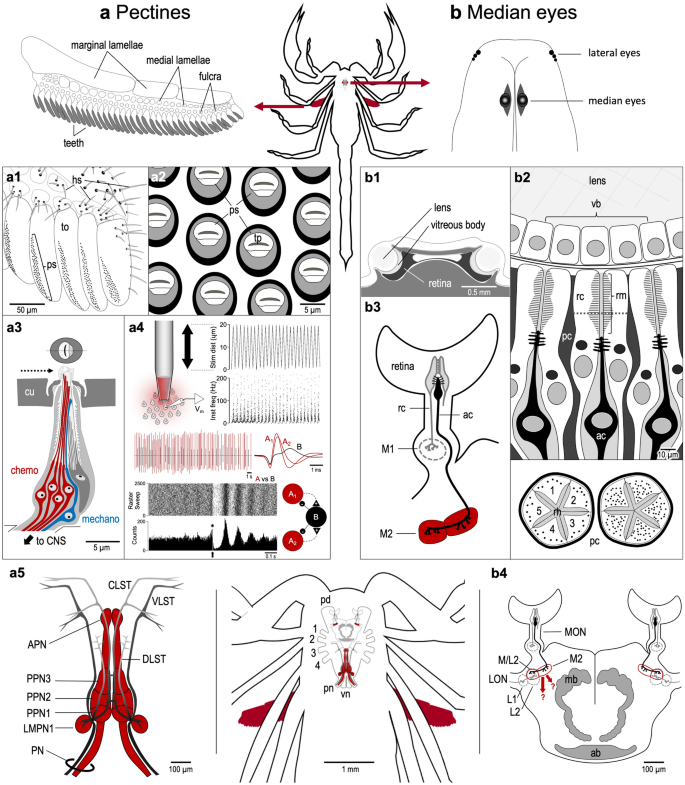The diagram is a highly detailed and annotated illustration of a scorpion, designed for educational or scientific purposes. The top section features a black and white image of a scorpion with its extended tail. Arrows point from this central image to the left and right. The left arrow, labeled with "A," indicates the pectines and details their structure with annotations such as teeth, fulcrum, medial lamella, and marginal lamella. The right arrow, labeled "B," points to the median eyes, also annotated with accompanying labels. Below the central image runs two columns, one under "A" and one under "B," each containing additional diagrams. These sub-diagrams are labeled sequentially as A1, A2, A3, A4 for the pectines, and B1, B2, B3, B4 for the median eyes, further detailing the scorpion's anatomy. The entire diagram is presented against a white background, making the intricate details and specialized annotations more legible and suited for in-depth study by those in the field of arachnology or related sciences.